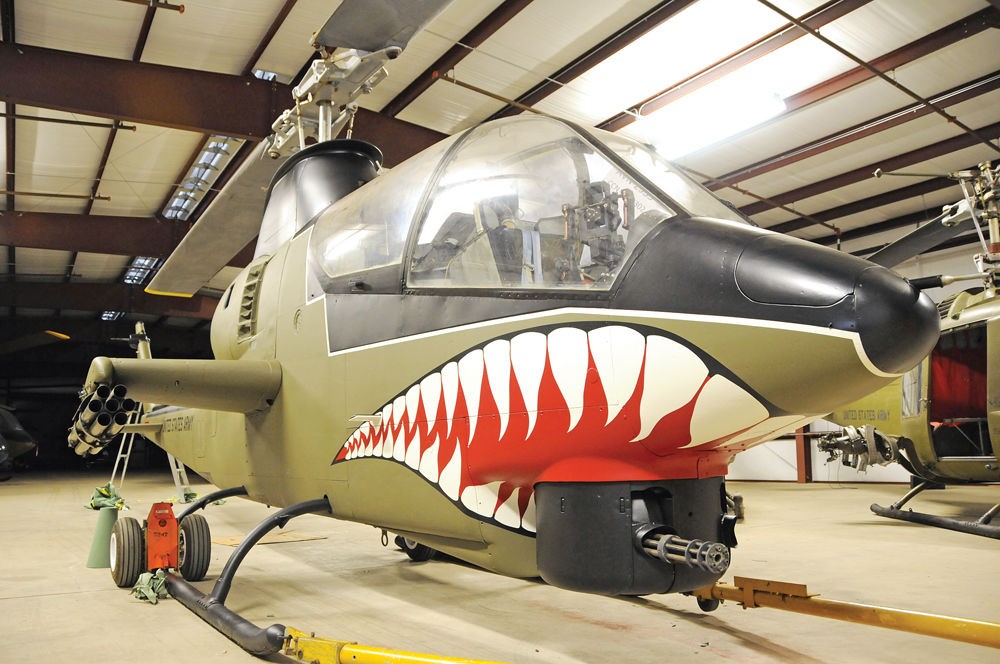Inside a large hangar with overhead black beams contrasted by white spaces, two helicopters are prominently displayed. The central helicopter, fully visible, features a striking design with a menacing mouth painted underneath. This graphic showcases sharp white teeth with a red background, accentuating its intimidating appearance. The body of the helicopter is predominantly tan with a black top, and its black propeller sits atop the fuselage. This military chopper, which appears to have olive green undertones, is outfitted with landing bars, small wheels, and a gun turret at the front, suggesting formidable firepower. Additionally, missile pods are mounted on its left side. The floor of the hangar is a tan color, matching the earthy tones of the helicopter. To the right stands a partially obscured helicopter, where only its door is visible. Meanwhile, the helicopter to the left is fully exposed, featuring small wheels, a ladder at the back, and some front attachments resembling pipes. This impressive scene captures the formidable essence and detailed designs of these helicopters amidst the structured yet simplistic hangar environment.